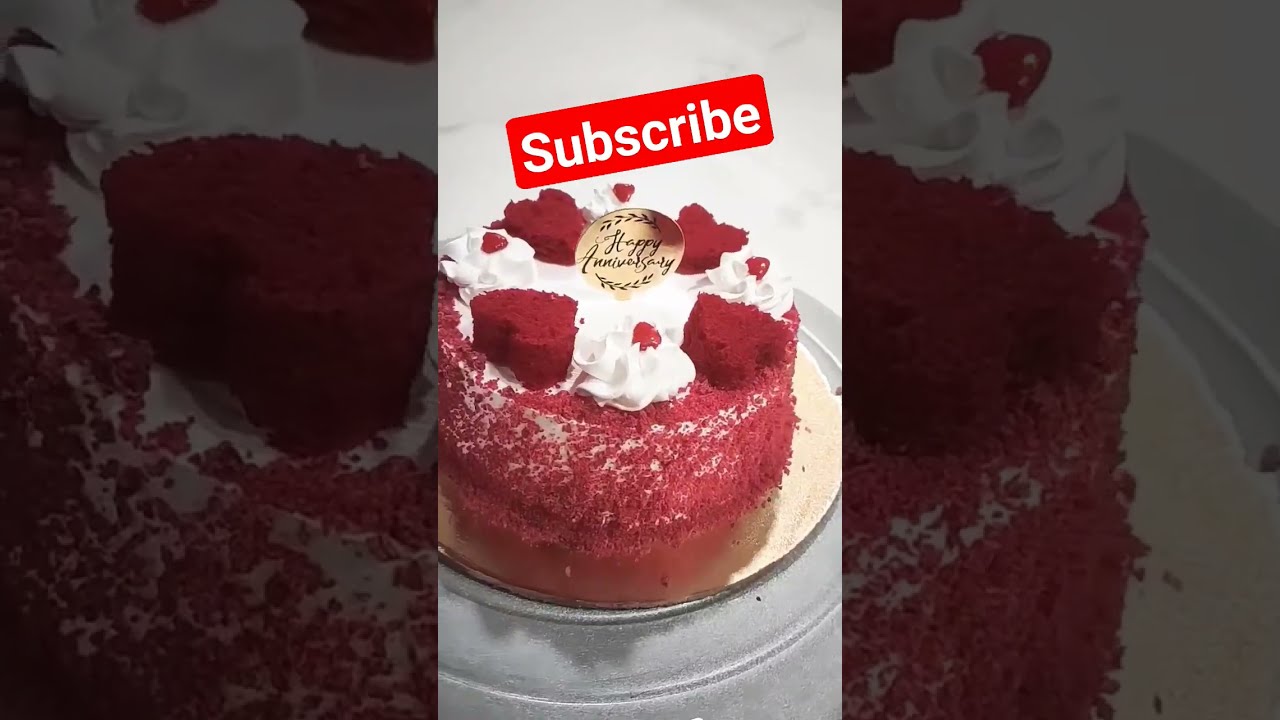The image features a beautifully crafted cake, prominently displayed in the center of a wide, horizontal photograph. The cake appears to be red velvet or strawberry shortcake, sitting elegantly on a dual plate arrangement—a circular gold plate atop a clear glass one. The cake is adorned with smooth white frosting and generously covered with reddish-maroon crumbs along its edges. Atop the cake, four heart-shaped pieces of cake, decorated with dollops of whipped cream, encircle the top. Between each heart are small, cherry-topped whipped cream swirls, complemented by cinnamon hearts. A gold plaque, inscribed with "Happy Anniversary" in black script and embellished with delicate leaf designs, sits prominently among the decorations. Above the cake, a red rectangular banner with rounded corners and the word "subscribe" in white letters is displayed, angled slightly to the right. The entire center image is layered on a darker, zoomed-in version of the same cake, forming an aesthetically pleasing and detailed backdrop.